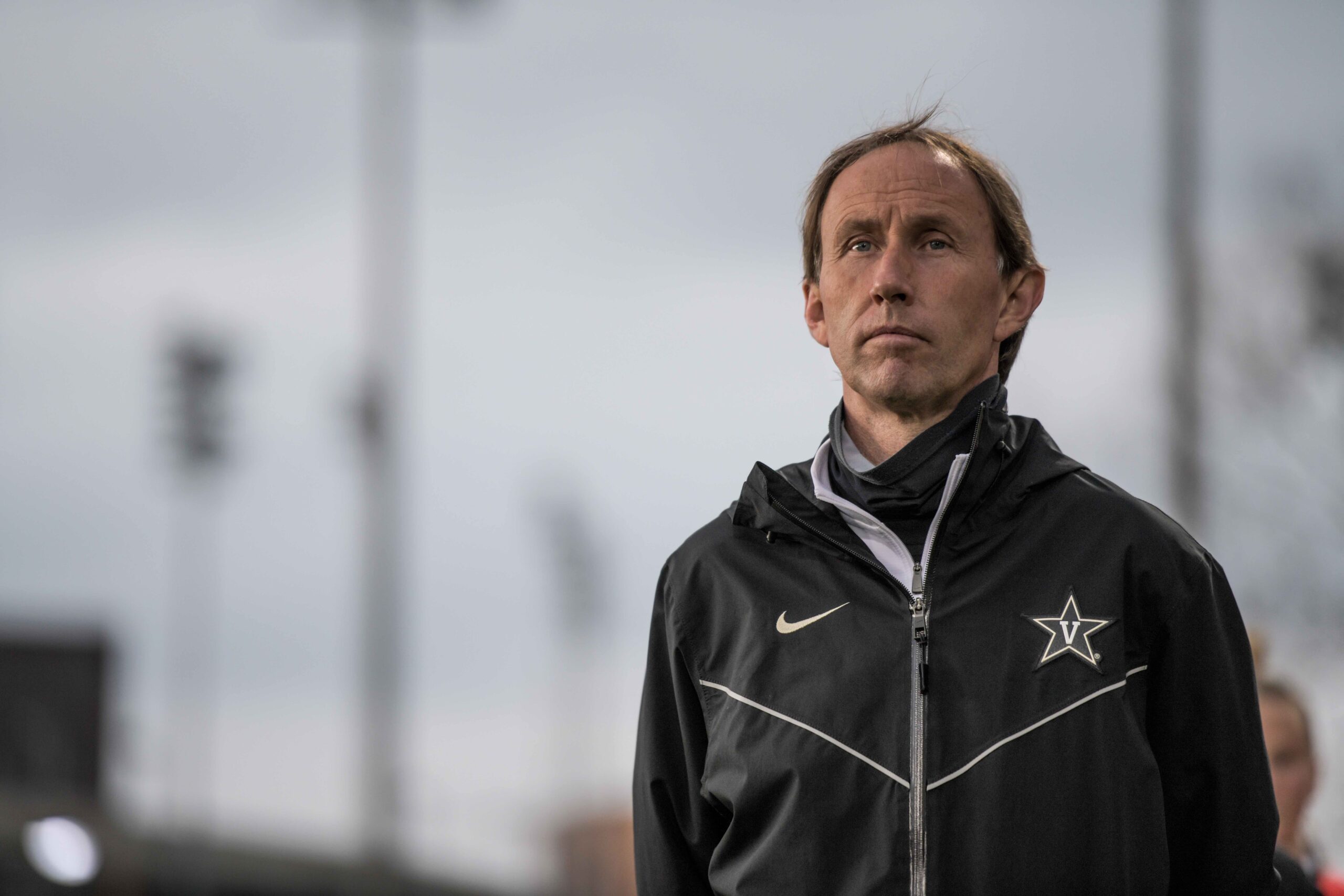This photograph captures a middle-aged man, possibly in his 50s, standing outdoors, seemingly in a stadium or on a sports field, as suggested by the tall poles with lights in the background. The image is predominantly gray with a blurry backdrop, emphasizing the man who stands slightly to the right of the center. He has brown hair and is wearing a black Nike zip-up jacket, possibly a wind or raincoat. The jacket features a white Nike swoosh on the right chest and a black and white star with a white ‘V’ on the left, indicating a potential affiliation with Vanderbilt. Underneath, he wears a black shirt. He also has a black face mask pulled down. His expression is neutral, and he is looking off into the distance. A partial image of another person is visible, blurry, behind his left shoulder. Only the upper part of his body is visible in the photograph.